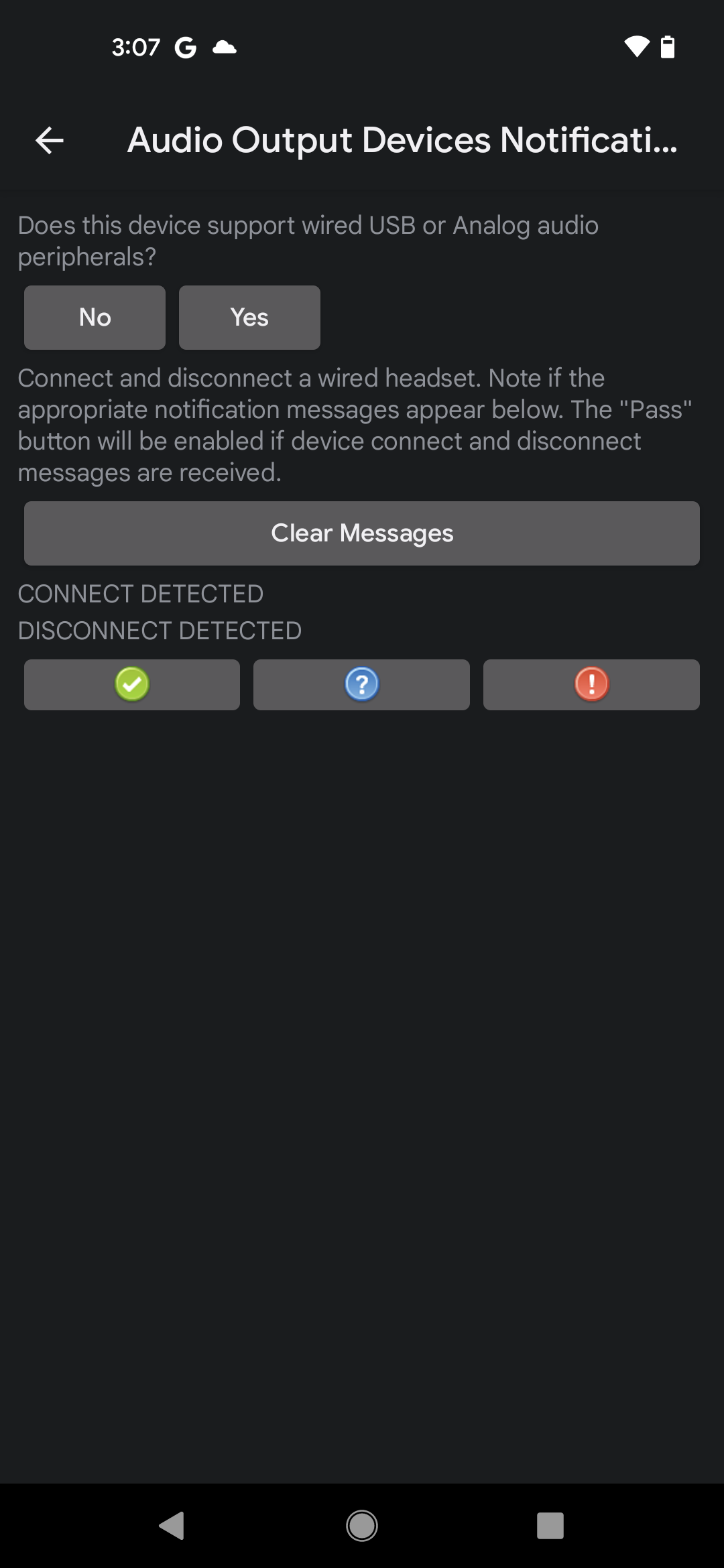The image displays the settings menu of a smartphone with a predominantly black background. At the top of the screen, the status bar shows the time as 3:47 PM, a cloud icon with the Google logo, Wi-Fi signal strength, and an almost full battery icon. 

The main menu is titled "Audio Output Devices Notification," with a left-facing arrow at the top left corner. Beneath the title, in gray text, it states, "Does this device support wired USB or analog audio peripherals?" Two gray boxes labeled "No" and "Yes" are provided for user selection.

Further down, gray text instructs, "Connect and disconnect a wired headset. Note: If the appropriate notification messages appear below, the pass button will be enabled if device connect and disconnect messages are received." Below this instruction, there's a gray box with white text labeled "Clear Messages."

At the bottom of the screen, under the instruction, a gray text status area indicates "Connect detected" and "Disconnect detected." Three indicator boxes are present: the first features a green checkmark inside a circle, the middle one has a blue circle with a white question mark, and the right one displays a red exclamation mark inside a circle.

At the very bottom of the screen are the navigation buttons typical of an Android device: a left arrow, a circle, and a square.